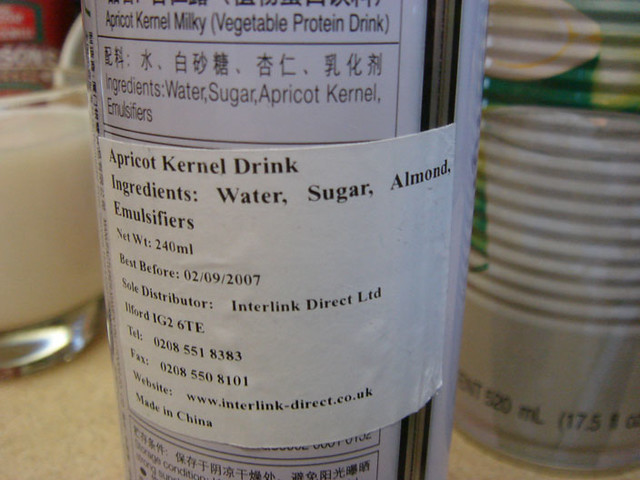This photograph, taken indoors on an off-white countertop, features a partially visible tall round can of a vegetable protein drink. The can is labeled predominantly in black text with Chinese characters and English. At the top, the can reads "Apricot Kernel Milky" followed by "Vegetable Protein Drink" in smaller black writing within parentheses. Below these, there are Chinese characters, succeeded by a list of ingredients: Water, Sugar, Apricot Kernel, Emulsifiers. A large square white sticker on the center of the can features black text detailing the product: "Apricot Kernel Drink," its ingredients (Water, Sugar, Almond, Emulsifiers), the net weight (240 milliliters), and expiration date (Best Before 02-09-2007). Additionally, it lists the sole distributor as Interlink Direct LTD located in Ilford, IG2-6TE, UK, along with contact information (phone: 0208-551-8383, fax: 0208-550-8101, website: www.interlink-direct.co.uk), and notes that it is Made in China. Adjacent to the can on the left is a small clear glass containing a whitish fluid resembling 2% milk. On the right, there is another tall ridged can with white, green, and black designs, accompanied by what looks like a plastic sleeve of small disposable bowls.